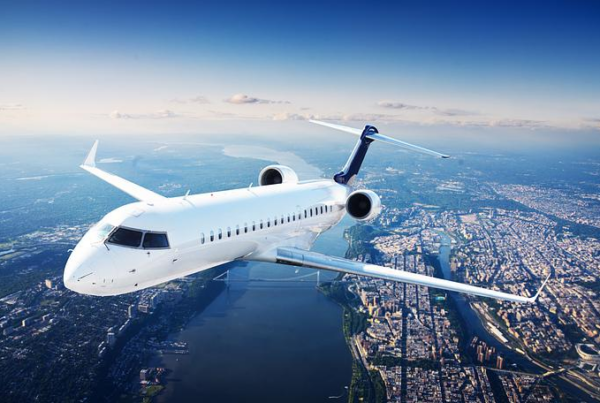The image captures a white passenger airplane with a blue tail in flight, viewed from a position seemingly in front and slightly above it, giving the impression that we are in another aircraft. The plane, which has approximately 15 windows along its fuselage and twin jet engines mounted at the rear, is flying over a sprawling urban landscape, identified as New York City. Below it, you can see a network of buildings, tiny houses, and notable landmarks like Yankee Stadium in the Bronx and possibly the George Washington Bridge. The airplane is positioned directly above the expansive Hudson and East Rivers, which flow into the background. The sky is a deep blue with a few scattered clouds.